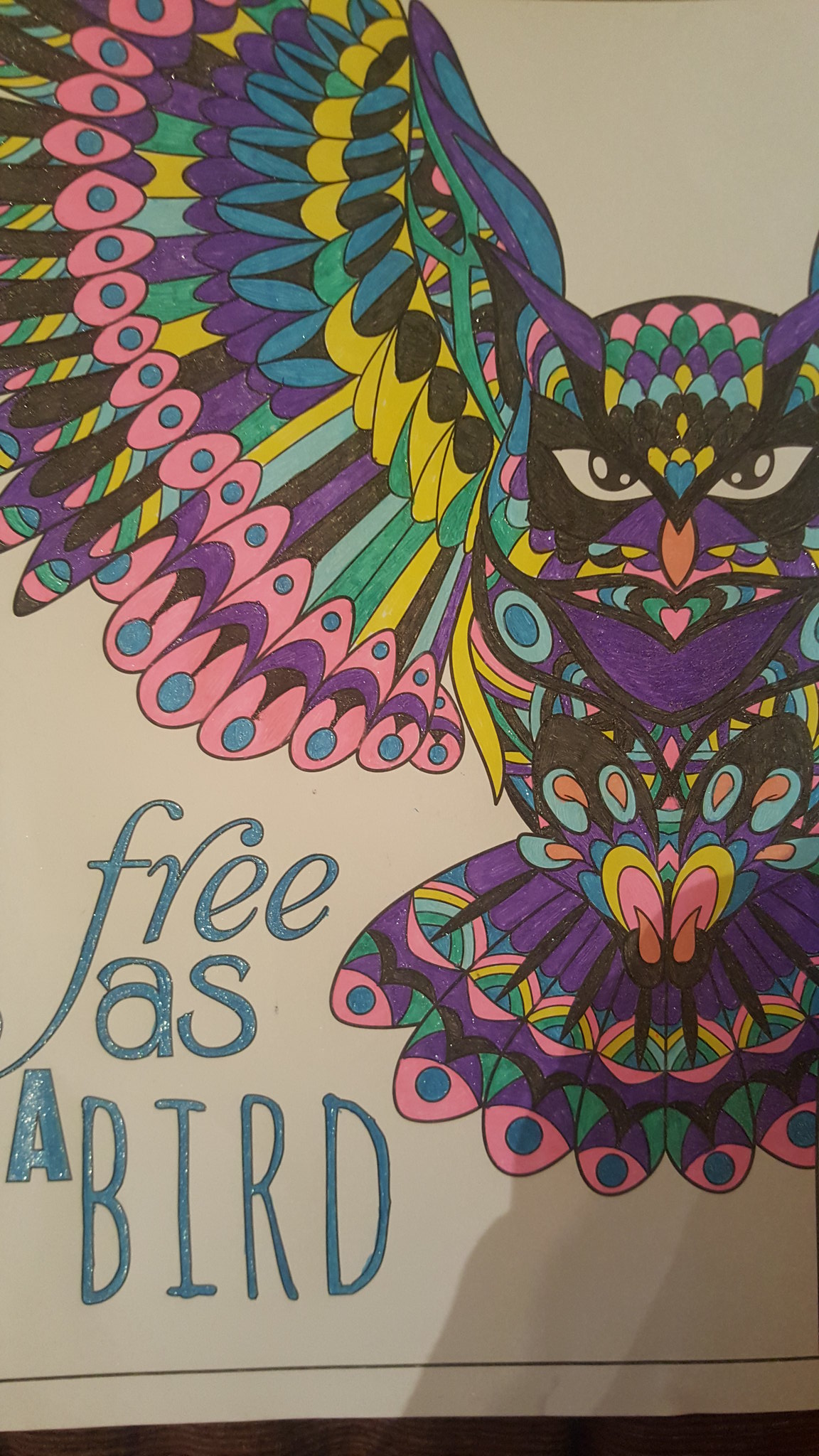This is a color photograph of what appears to be a page from an adult coloring book. The white page features a meticulously detailed owl in flight, with the body aligned to the right side of the image and a partially outstretched wing extending upwards and to the left. The intricate owl illustration is divided into many geometric shapes, filled with a vibrant palette of colors — predominantly purples and pinks, with accents of yellow, green, blue, light blue, black, and orange. The eyes of the owl are strikingly left uncolored with black pupils, giving it an intense, focused gaze directed at the viewer. At the bottom left corner of the image, the text "Free as a Bird" is written in different fonts — cursive, serif, and sans serif — and colored in a light blue or turquoise hue. The overall background is white, and there’s a subtle shadow cast over the bottom right corner from an unspecified source, adding depth to the tall, narrow composition.